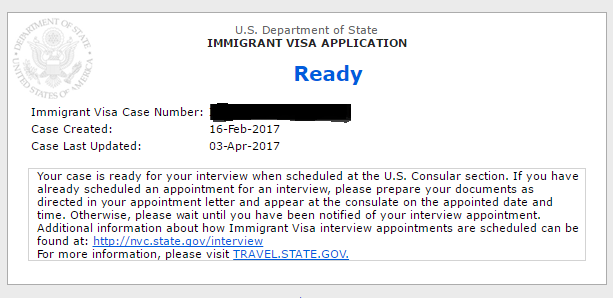This is a detailed screenshot depicting an individual's immigrant visa application status for the United States. In the upper left corner, the emblem of the U.S. Department of State is visible, featuring the iconic eagle clutching arrows and an olive branch, though it appears slightly grayed out against a pink background. The primary content is presented on a white field bordered by a simple 1-pixel gray outline. 

At the top center, bold text states "U.S. Department of State Immigrant Visa Application," followed by large blue text reading "Ready." The immigrant visa case number is conspicuously blacked out for privacy.

To the left, beneath the emblem, important details are listed: "Case Created: 16 February 2017," and "Last Updated: 3 April 2017." 

A notification in a bordered text field informs the applicant that their case is ready for an interview at the U.S. consulate. The message advises, "If you've already scheduled an appointment for an interview, please prepare your documents as directed in your appointment letter and appear at the consulate on the appointment date and time. Otherwise, please wait until you have been notified for your interview appointment." Further guidance directs readers to the URL “http.nvc.state.gov/interview” for additional information regarding interview appointments and to “travel.state.gov” for more general queries, with the latter link prominently underlined in blue capital letters.

This structured and detailed view provides clear instructions and status updates, ensuring the applicant is well-informed about the next steps in their visa application process.